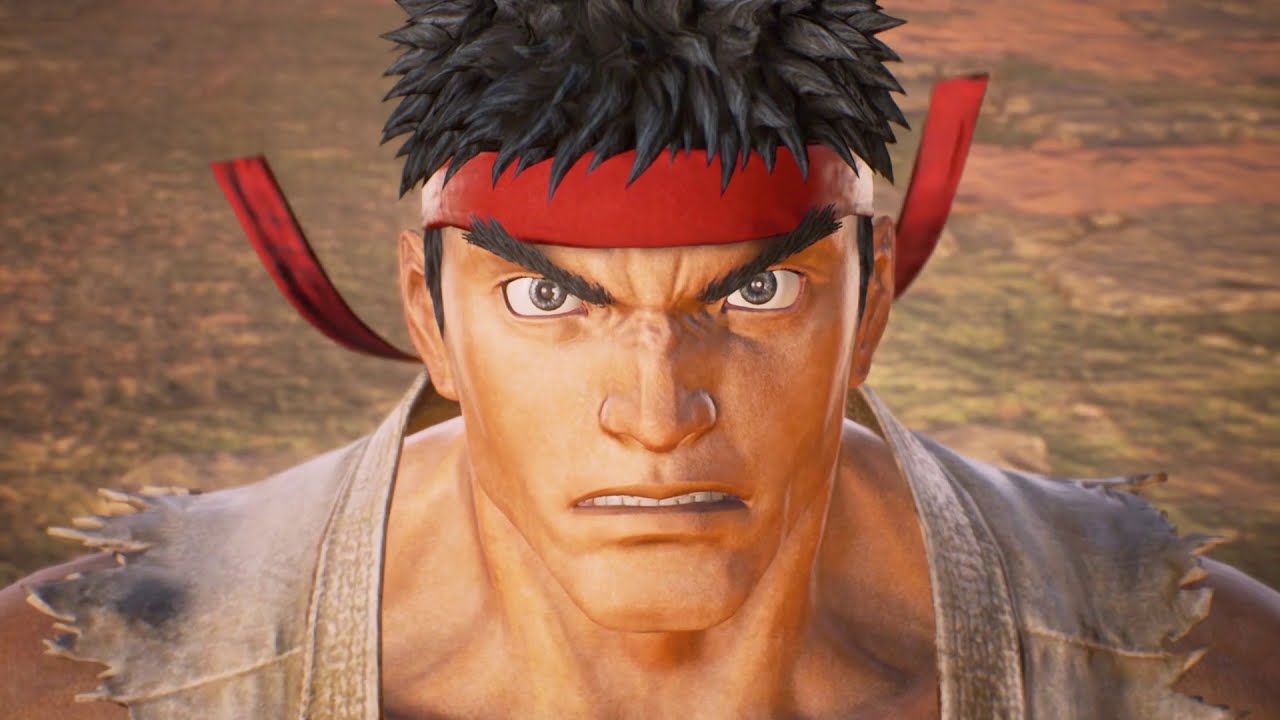The image is a detailed close-up of a cartoon or video game character, identified as Ryu from Street Fighter. The character is centered in the frame, viewed from the shoulders up, with a fierce and angry expression. His black, short, and spiky hair is complemented by a red headband tied around his forehead, with the straps visibly tied at the back and waving slightly. Ryu’s eyebrows are sharply pointed downwards in a V shape, enhancing his menacing gaze, which is directed straight ahead through his gray eyes. His nose is scrunched up, further emphasizing his anger, and his mouth is slightly parted, revealing clenched teeth. His face is thin and chiseled. He’s clad in a white karate uniform with the sleeves torn off jaggedly, showing signs of wear and dirt. The background is a somewhat ambiguous mix of dirt, rocks, and sparse light green grass, painted in muted green and brown tones, reinforcing the rugged and intense atmosphere of the scene.